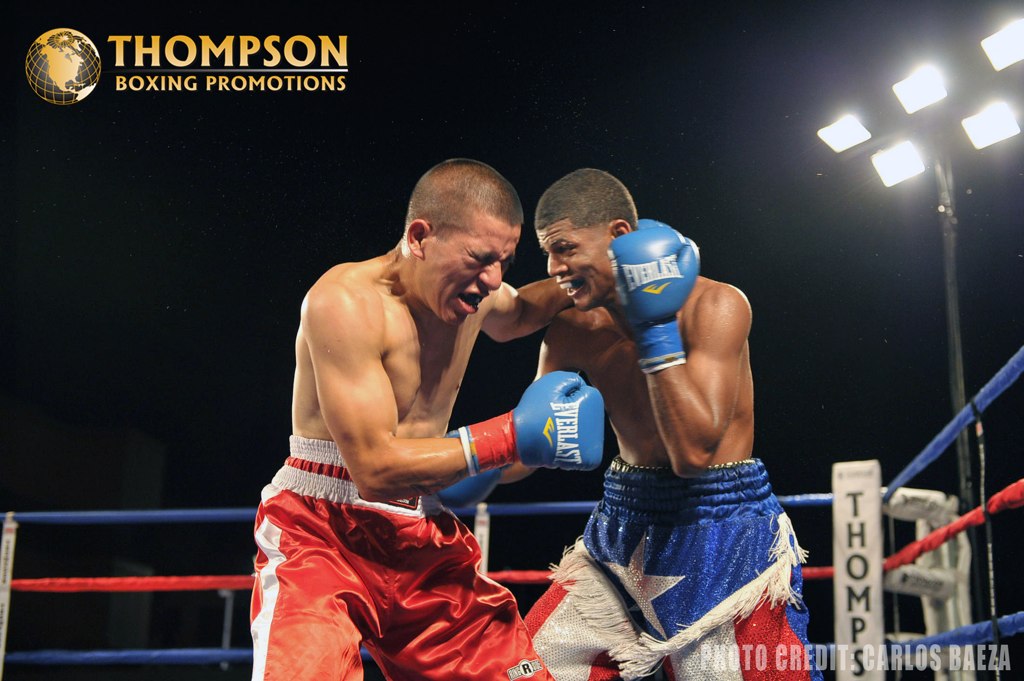The image captures an intense boxing match between two fighters, both centered in the ring and facing each other. One fighter is dressed in red and white shorts with red tape on their blue Everlast gloves, while the other dons red, white, and blue shorts featuring silver stars, with blue tape on their matching blue Everlast gloves. The ring is framed with blue, red, and blue ropes with white ends, featuring subtle black text. Overhead, floodlights shine brightly, illuminating the scene against a dark, black backdrop. In the top left corner, the gold globe logo of Thompson Boxing Promotions is visible, while the bottom left corner credits the photographer, Carlos Baeza. This indoor setting, likely a stadium, showcases the dramatic atmosphere of the boxing match.